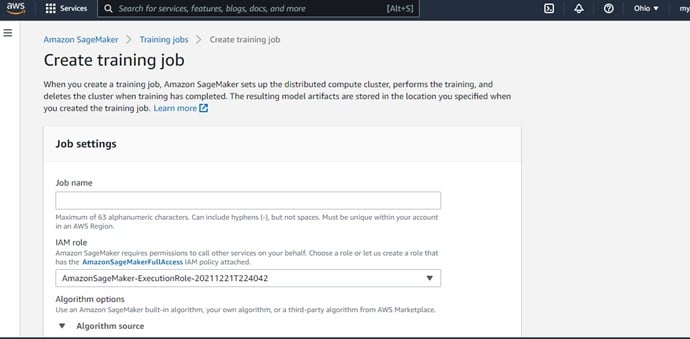The screenshot displays a webpage from the AWS (Amazon Web Services) site. At the top is a horizontal, charcoal black navigation bar. On the far left of this bar is the AWS logo in white font, followed by Amazon's recognizable yellow, rightward-facing arrow. Adjacent to the logo, there's a cluster of small white circles with the word "Services" written in white font.

To the right of the "Services" section lies a search field, identifiable by a white magnifying glass icon. The placeholder text in this field reads, "Search for services, features, blogs, docs, and more," with a note within brackets indicating the shortcut (Alt + S).

On the upper right corner of the toolbar, there are three icons: a bell for notifications, a circle with a question mark symbolizing help or support, and a drop-down menu labeled "Ohio," presumably indicating the selected AWS region.

Below the black navigation bar is a light gray webpage featuring Amazon SageMaker. The headline reads "Amazon SageMaker," followed by a breadcrumb trail with arrows indicating the navigation path: "training jobs" > "create training job" - with the latter option being selected. The main body text explains, "When you create a training job, Amazon SageMaker sets up a distributed compute cluster, performs the training, and deletes the cluster when training has completed."